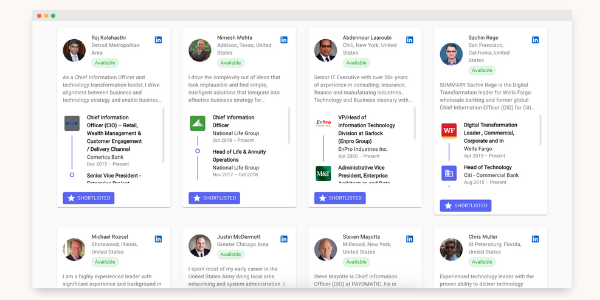The image depicts a webpage, possibly an employee directory or search results, showcasing eight individuals. Their roles seem to be related to information technology and digital transformation within various organizations. Here is a detailed breakdown from left to right:

1. **Name**: [Unclear, possibly Kaj Kaleski]
   - **Location**: Detroit Metropolitan Area
   - **Position**: Chief Information Officer, Retail Wealth Management
   - **Availability**: On LinkedIn
   - **Details**: Although the text is slightly blurred, Kaj appears to be a seasoned CIO with expertise in technology and retail wealth management.

2. **Name**: Makesh Mehta
   - **Position**: Chief Information Officer
   - Other specifics are obscured, but analogous to Kaj, Makesh likely holds a critical IT leadership role.

3. **Name**: [Unclear]
   - **Location**: New York
   - **Position**: Vice President, Head of Information Technology
   - Details about this individual are blurry, but he holds a VP-level IT position indicating significant responsibility in managing technology operations.

4. **Name**: Sachin Raise (?)
   - **Location**: San Francisco
   - **Position**: Digital Transformation Leader
   - Sachin appears to drive digital innovation and change, a pivotal role in modernizing business processes.

The bottom row includes:
5. **Name**: Michael Rousset
   - **Location**: St. Petersburg
   - Photo suggests a professional attire, possibly indicating seniority.

6. **Name**: Justin McDermott
   - **Location**: New York (specific area blurry)
   - Shown with a formal look, possibly reflecting a high-ranking position.

7. **Name**: Steven [Surname Unclear]
   - **Location**: Greater Chicago Area
   - Details truncated, but appears professionally dressed.

8. **Name**: Chris [Surname Unclear]
   - **Location**: Illinois
   - Similar to the others, professionally attired with a summary cut off.

Overall, the page lists these eight professionals, providing partial insights into their roles, locations, and LinkedIn availability, with the first four providing more comprehensive information compared to the partially visible details of the latter four.